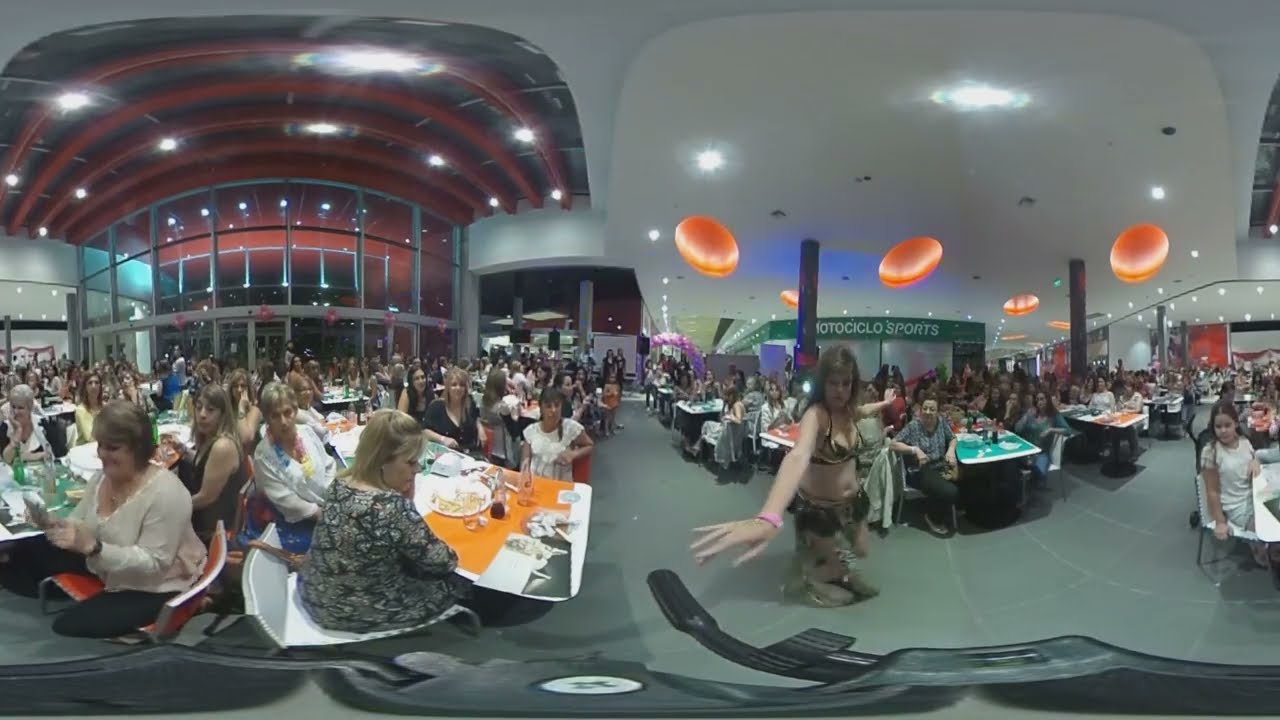In the forefront of the image stands a woman with short brunette hair, dressed in a green print bikini top and a long skirt, complemented by a pink bracelet on her right wrist. She faces forward, appearing to reach for something with her right hand while her left hand extends backward towards a substantial audience, predominantly women, who are seated at tables. The setting resembles a vast indoor venue, possibly an auditorium or a large cafe, filled with over a hundred people. There are noticeable large, round, orange light fixtures hanging from the white ceiling, which appears slightly curved. To the left, glass doors with a red semicircular rooftop and large windows and awnings are visible. A tent labeled "Moto Chiclo Sports" is set up in the back, suggesting some sporting convention or event. The audience is attentive, focused on the woman, indicating she is likely speaking or presenting to the crowd.